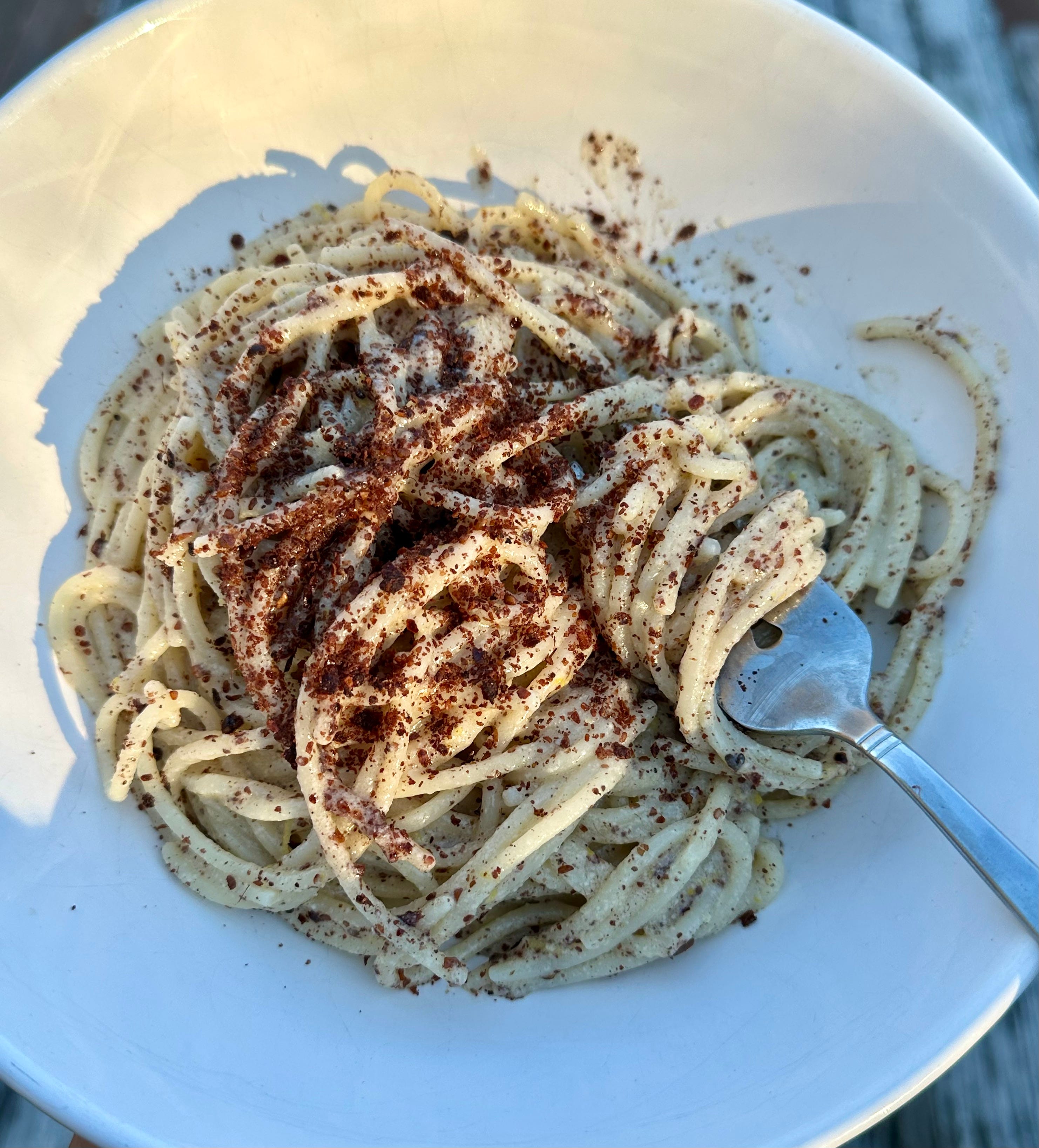The image depicts an overhead view of a dish, prominently featuring a white plate, which dominates the majority of the frame. The plate sits on what appears to be a gray wooden surface, likely a table, giving the impression of an outdoor setting bathed in natural sunlight. The illumination is more pronounced on the upper left side of the plate, casting shadows towards the lower right.

In the center of the plate is a pasta dish with thin noodles resembling linguine or spaghetti. The noodles are light in color, suggesting they might be tossed in a subtle sauce, and appear soft and tender. Sprinkled generously over the pasta is a reddish-brown seasoning, potentially paprika or a similar spice blend, concentrated heavily at the center and scattering towards the edges.

A silver fork enters the scene from the right, reaching across to the left, with noodles twirled around its tines, indicating that someone is in the process of eating. The meticulous details, such as the fork's positioning and the shadows cast by the pasta and utensil, enhance the sense of depth and texture in the image.